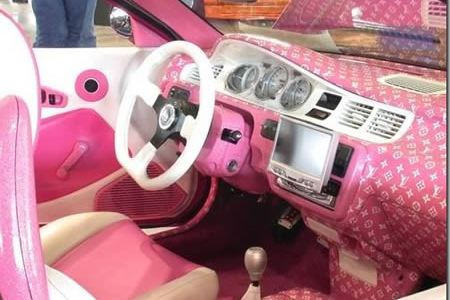This is a detailed photograph of a customized car interior, predominantly in pink and white. The image, taken indoors with artificial light, is horizontally rectangular with a thin gray border on the right side. It appears as if the photo was captured from the passenger seat, looking towards the dashboard and steering area. The driver's seat is fashioned in pink and white, matching the rest of the car's thematic design. 

The steering wheel and the dashboard area housing the gauges are white, contrasting with the pink body of the dashboard itself, which features a repeating white Louis Vuitton pattern. This pattern consists of the overlaid letters "L" and "V" along with various geometric stars and shapes. The center console, including the gear shift, is predominantly pink. 

On the right side, there is a display screen, possibly for GPS, and several air vents. The left side door panel is similarly pink and white, equipped with a pink crank for the window. Through the driver's side window, part of the outside is visible, including a pair of legs in blue jeans, indicating someone standing nearby. The overall whimsical design evokes a sense of a Barbie-inspired car interior, combining playful luxury with detailed craftsmanship.